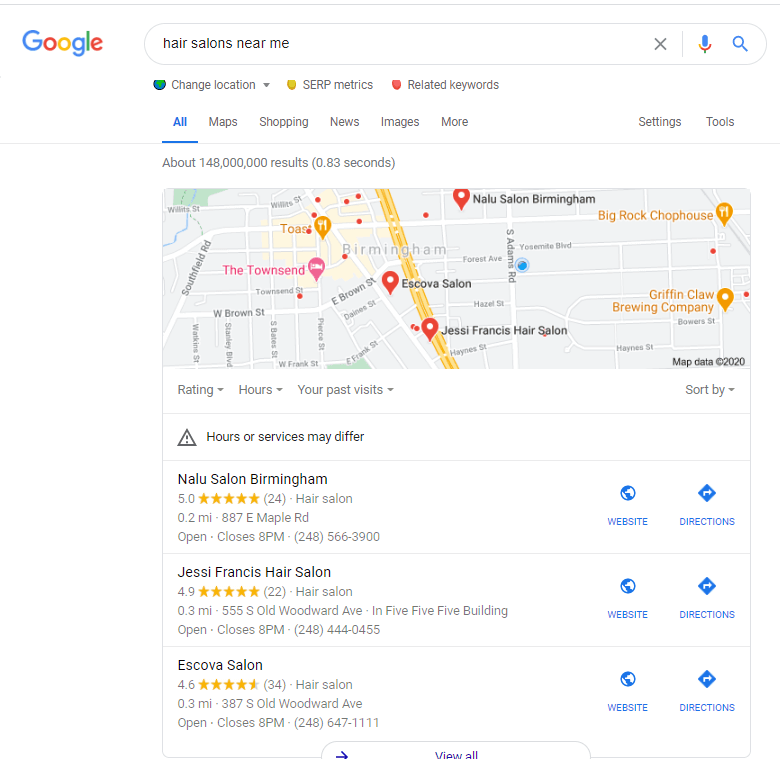This image is a cropped screenshot, potentially from a desktop, laptop, or tablet computer, displaying a Google search results page. The interface dimensions suggest it may not correspond to a usual desktop but are too large for a typical mobile phone, suggesting it could be from a tablet or a cropped desktop view. 

The screenshot captures the Google homepage, characterized by its clean, white background. In the upper-left corner, the iconic Google logo is displayed, with the individual letters colored in blue, red, yellow, blue again, green, and red, respectively. Below the logo is a long search bar extending across the screen, where the query "hair salons near me" has been typed.

Under the search bar, the usual navigational tabs appear, including "All," "Maps," "Shopping," "News," "Images," and "More," alongside options for "Settings" and "Tools." In this instance, the "All" tab is selected, leading to a display which includes a partial view of Google Maps. This map highlights nearby hair salons with red location pins, indicating their positions.

Additionally, the search results list three hair salons in a sequential order underneath the map section. Each listing provides comprehensive information, including star ratings, website links, directions, and contact details, facilitating easy access and comparison for the user.